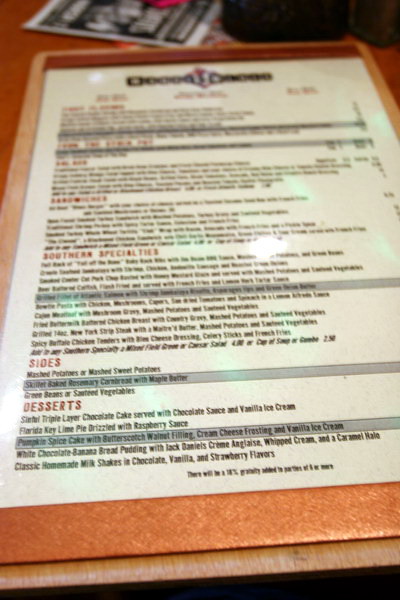The image is blurry and out of focus, making it challenging to decipher the text on the paper. The background features a reddish-brown wooden surface, likely a table. In the upper left corner, there's a white piece of paper with a black and red image on it. The upper right corner of the photo contains a vague, indistinguishable black object. The central focus is a light brown, golden-hued wooden menu board. At the top of the menu, an illegible name is displayed in bold black letters, followed by red text underneath. The menu includes a series of alternating paragraphs in black and red writing. Some of the black paragraphs have gray lines striking through them. Toward the bottom, there is a section labeled "Desserts" in red, followed by more black text with gray lines through it.